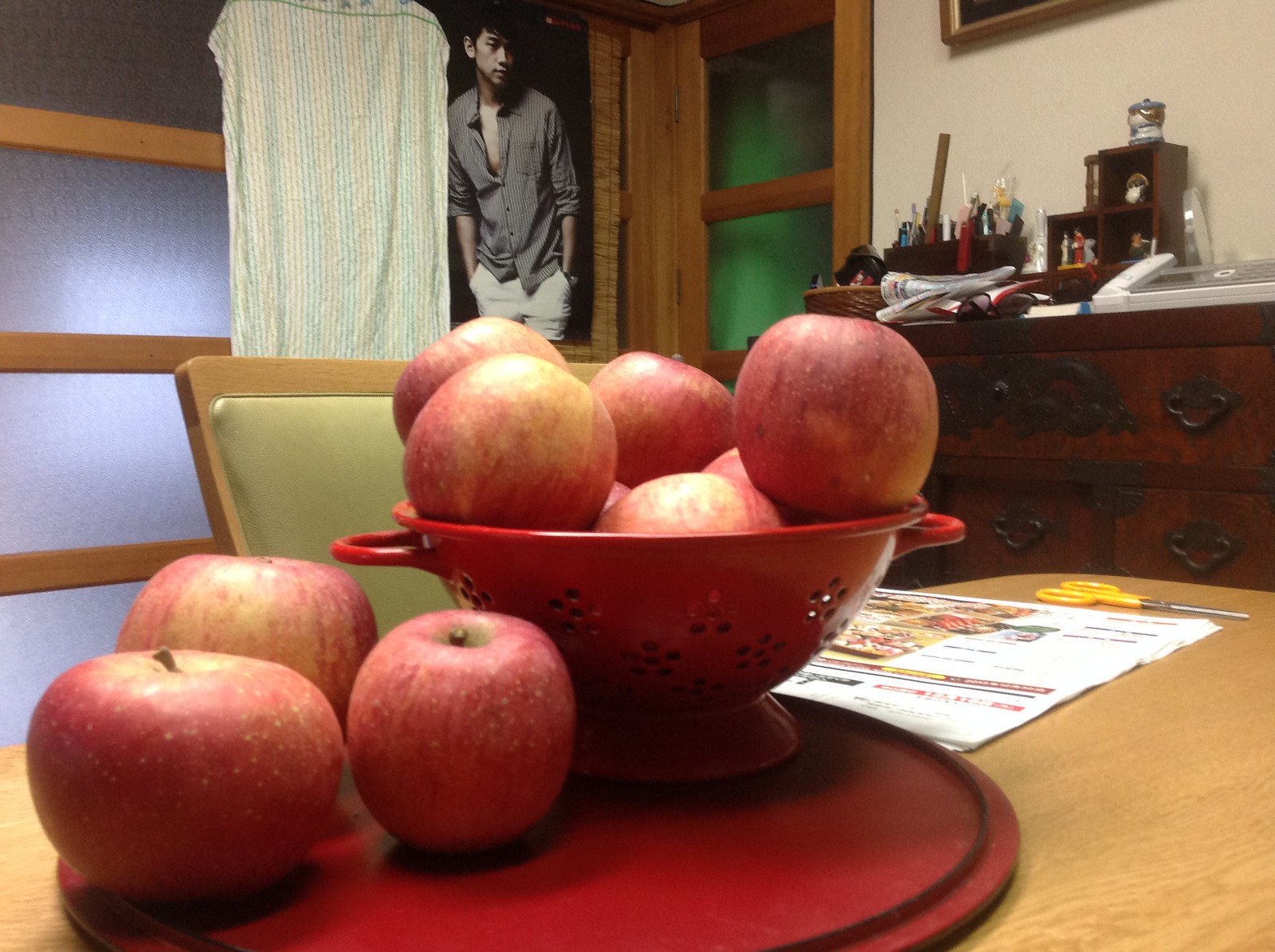The photograph captures a detailed scene of a cozy dining room. At the center, there's a wooden table adorned with various items. A striking red colander, perforated with holes and equipped with handles, serves as a fruit bowl filled with a mix of predominantly red and some green apples. This colander is positioned on the edge of a larger red tray alongside three loose apples of the same variety. Spread out behind the apples on the table is a newspaper with an orange-handled pair of scissors, suggesting an intent to cut something out. Directly behind the table, a wooden chair with a green padded backrest is visible, adding a touch of color and comfort to the scene. 

In the background, a smoked glass window, allowing light but obscuring details, provides a glimpse into another illuminated space. On the opposite side of the table stands a dark wooden dresser adorned with ornate handles, cluttered with various indistinguishable items, enhancing the room's lived-in feel. A closed door with brown panels is also visible, with a man dressed in a gray shirt and white pants casually standing beside it, hands in his pockets. Additionally, a white shirt with stripes hangs on the wall to the side, contributing to the cozy and personal atmosphere of the room.